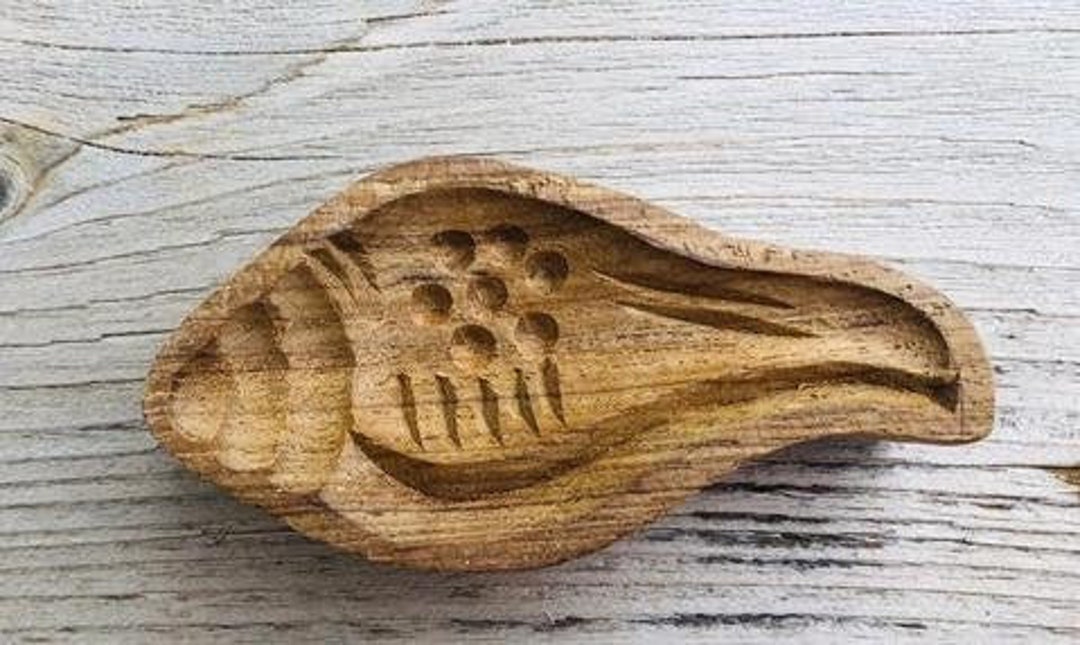This image showcases a detailed wooden art piece, possibly a functional item like a spoon rest or decorative wall piece, shaped intriguingly like a conch shell. The piece is a lighter brown in color and carved with intricate, rustic patterns. Distinguishing features include a series of seven circular indentations in the center, reminiscent of the top spirals of a seashell. Below these circles are vertical lines, adding texture and complexity. Additionally, a squiggly, swirly line runs along the length of the shell, extending from the center towards the thinner, right side of the piece. This art piece rests on or is photographed against a lighter, white wooden surface with black or beige cracks, creating a backdrop that contrasts and highlights the craftsmanship and detail of the wooden shell. The overall composition highlights the artistic and potentially functional qualities of the piece, reflecting its archaic charm with modern rustic aesthetics.